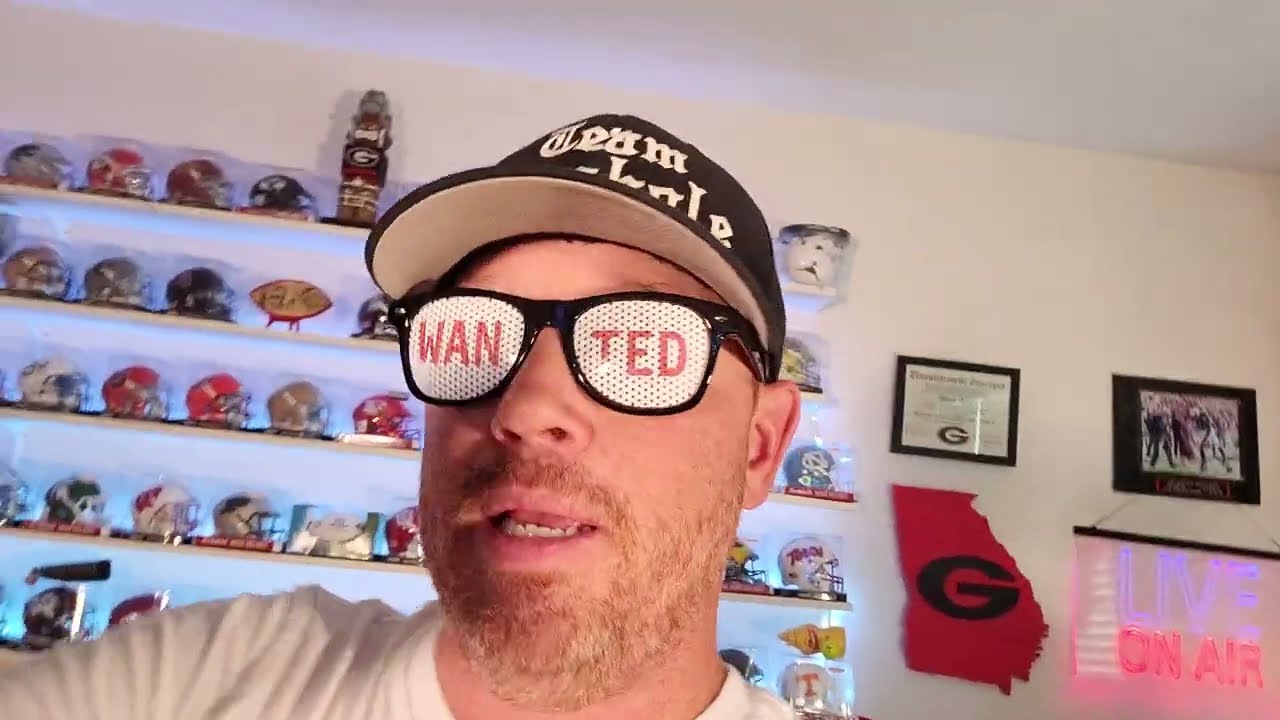This image is a selfie of a man with light brown stubble forming a goatee. He’s wearing a black cap with partially obscured text and black costume glasses featuring white lenses that spell out "WANTED" in red font, with "W A N" on the left lens and "T E D" on the right. The man is standing in front of a beige wall decorated with several white shelves, all backlit with blue lighting, displaying an array of small football helmets in various colors, including red, silver, black, green, and multiple shades of blue, suggesting he is a collector. To the right of the shelves, there is a framed object—possibly a photo or certificate—featuring a red silhouette of the state of Georgia with a large black "G" on it. Below it, there is another picture frame containing the phrase "ON AIR" in purple and red font.